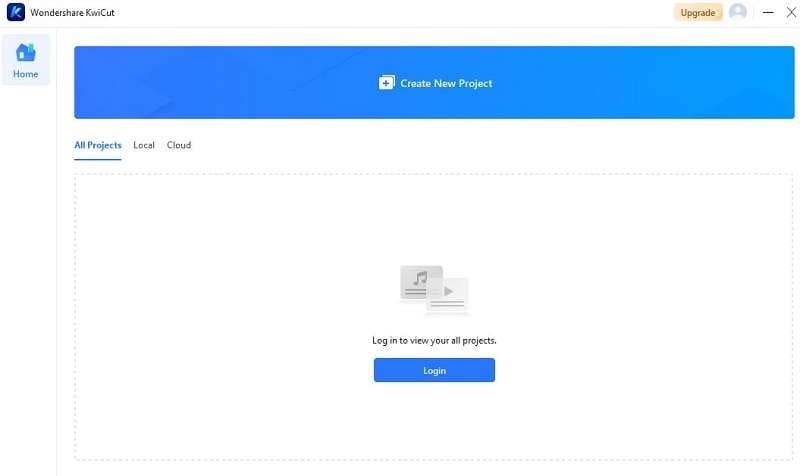The website displayed has a predominantly blue color scheme, featuring a navy blue background with various graphic elements. In the upper left-hand corner, there is a logo, albeit somewhat indiscernible, consisting of a navy blue base with a lighter blue shape inside. Adjacent to this logo, the words "Wondershare Kwikut" are prominently displayed, with a stylized capital 'K', 'W', and 'C'.

On the upper right-hand side of the webpage, there is an 'Upgrade' button, accompanied by an option to upload a picture or avatar, along with minimize and close icons.

Directly beneath the Wondershare Kwikut logo on the left, there is a 'Home' link. Spanning across the top of the page is a large blue banner, notable for containing a plus button labeled 'Create New Project.'

Below this banner, users are presented with three project view options: 'All Projects,' 'Local,' and 'Cloud.' 'Local' presumably refers to projects stored on the user's computer, 'Cloud' to those saved in the cloud, and 'All Projects' encompassing both.

The center of the webpage features a vast white workspace. Within this area, there are icons indicating different content types: a rectangle with music notes, and another with a play symbol. Additionally, there is a prompt instructing users to 'Log in to view all your projects,' accompanied by a conspicuous blue 'Log In' button.